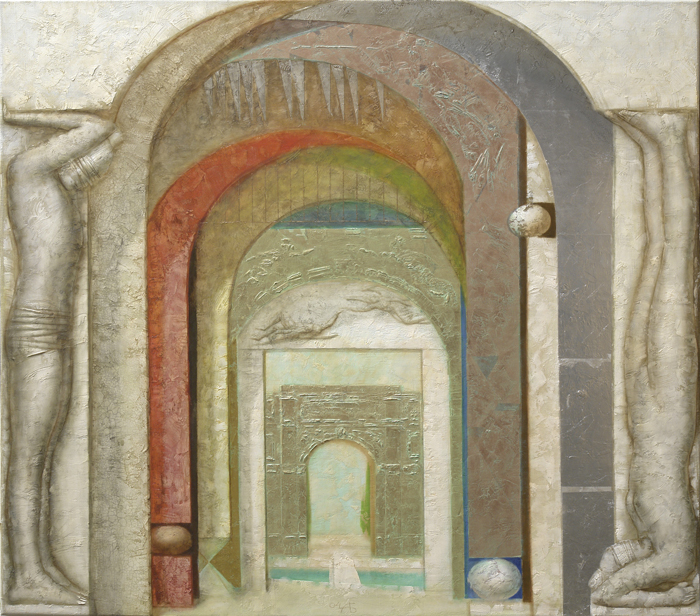The image depicts a meticulously detailed painting of a series of nested arches leading down the center, with no associated text. The first arch in the foreground features a brown and silver design, followed by a purely brown arch. Next, there's an orange archway, followed by a green one, creating a sense of depth and progression. On each side of the foreground arch stand two stone-like sculptures of men; the statue on the left stands upright with its hands bent upwards above its head, while the statue on the right is positioned upside down, mirroring the pose. The overall color palette includes tones of white, tan, brown, orange, turquoise, gray, and off-white. This artistic composition blends stone textures with vibrant colors to create a visually intriguing and well-thought-out piece of artwork.